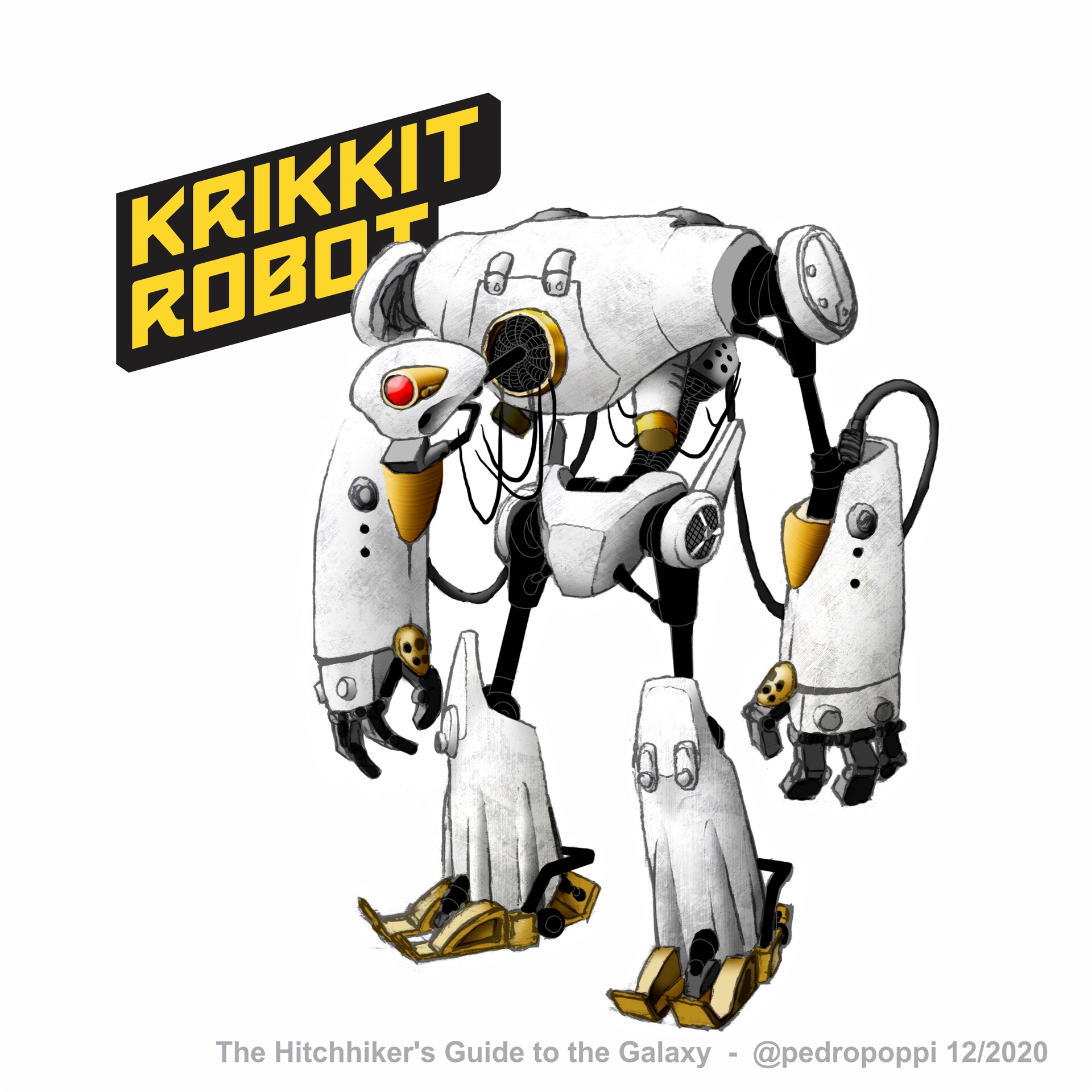This is a detailed cartoon drawing presenting a distinctive robot. In the upper left corner, large yellow letters spell out "Krikkit Robot" with a black box behind the text. Central to the image is a largely white robot, headless, with intricate design details including black connecting joints at its limbs. Highlighting its somewhat human-like posture, the robot appears to be hunched over, with arms extending down to its knees. The chest, a central focal point, features a gold circle with an internal black circle, a protruding small black pole, a distorted white round shape resembling an eye with a red dot, and a gold piece resembling a beak hanging below. Additional gold elements are on the neck collar, parts of the arms, and toes. Connected from the back, wires lead towards its arms, which have three fingers and a thumb each. Below the robot in light gray text, it reads "The Hitchhiker's Guide to the Galaxy at Pedro Papi 12, 2020."